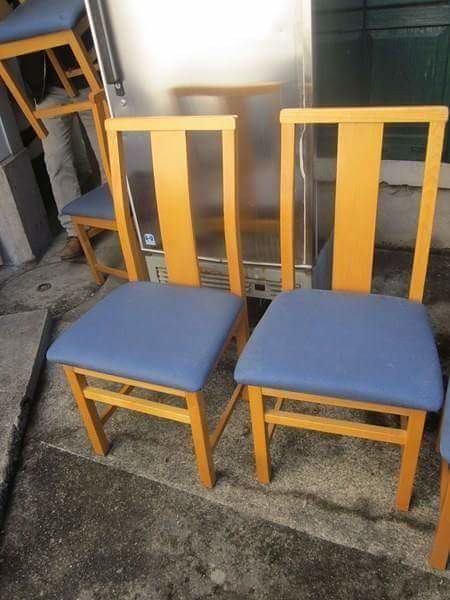This image showcases two light-colored wooden chairs with blue, form-fitted cushion seats. Each chair features a backrest with three vertical sections—a centerpiece flanked by two side pieces, connected by a top horizontal bar. They have slats between the legs for added stability. The chairs are situated on what appears to be cement flooring in a storage or basement-like area. Behind them stands a stainless steel refrigerator, reflecting one of the chairs on its surface. To the right of the fridge, there are two more identical chairs, one on the floor and the other seemingly suspended above it. Additionally, part of the scene includes the legs of a man wearing khaki pants and boots, partially visible with a black coat, carrying one of the chairs. In the background, there is a green wall and a dark window in the upper right corner, adding to the industrial atmosphere of the setting.